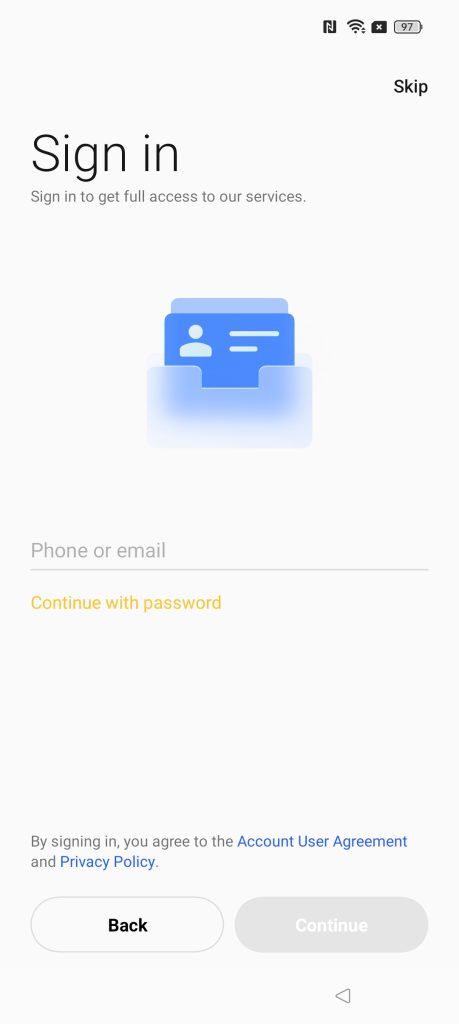The image is a screenshot of a smartphone screen in a vertical orientation with a white background. At the top right corner of the screen, there are several icons in black, including the Wi-Fi icon, battery charge icon, and other unidentified icons. Below these, the word "SKIP" is displayed.

The screen shows the sign-in landing page for an unspecified service. At the top left, the heading "SIGN IN" is written in large letters, with the 'S' capitalized. Directly below this, in smaller font, it states "Sign in to get full access to our services." The text is in black or gray.

Beneath the text, there's an illustration of a translucent file drawer or inbox-shaped object. Inside this, there is what appears to be a blue identification card featuring a white circle on top of a hill-shaped figure representing a person. The card includes two longer white lines and a short white line intended to represent text.

Further down the screen, there's a blank area followed by a thin, faint gray line extending across the width of the screen. Above this line, it says "Phone or Email," indicating where users should enter their information. Below this line in orange text, it reads "Continue with Password."

Another blank white space follows, leading towards the bottom of the screen where there's text stating, "By signing in you agree to the Account User Agreement and Privacy Policy." The phrases "Account User Agreement" and "Privacy Policy" are in blue, indicating they are clickable links for further details.

At the bottom of the screen, there are two oblong buttons. The left button is labeled "BACK" in bold black text with a gray outline, while the right button is labeled "CONTINUE" in white text on a solid gray background. Below the "CONTINUE" button, there is a left-pointing triangular arrow icon.